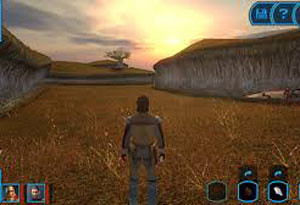In this low-resolution still from a video game, we see the back of the main character centrally positioned at the bottom of the frame. The character, distinguished by dark brown hair, is wearing a long-sleeved brown shirt and jeans, with what appears to be a belt carrying guns. The setting features the character standing amidst brown and green grass, flanked on both sides by gray and light green rocky walls or cliffs. The horizon reveals a picturesque hill with a single tree, set against a dramatic sky transitioning from golden hues to pink and gray, hinting at a sunset or sunrise. Decorated with game interface elements, the screen shows two character squares in the lower-left corner and three in the lower-right corner, while the upper right includes a square with a smaller square inside of it and another square with a question mark, enhancing the digital ambiance.